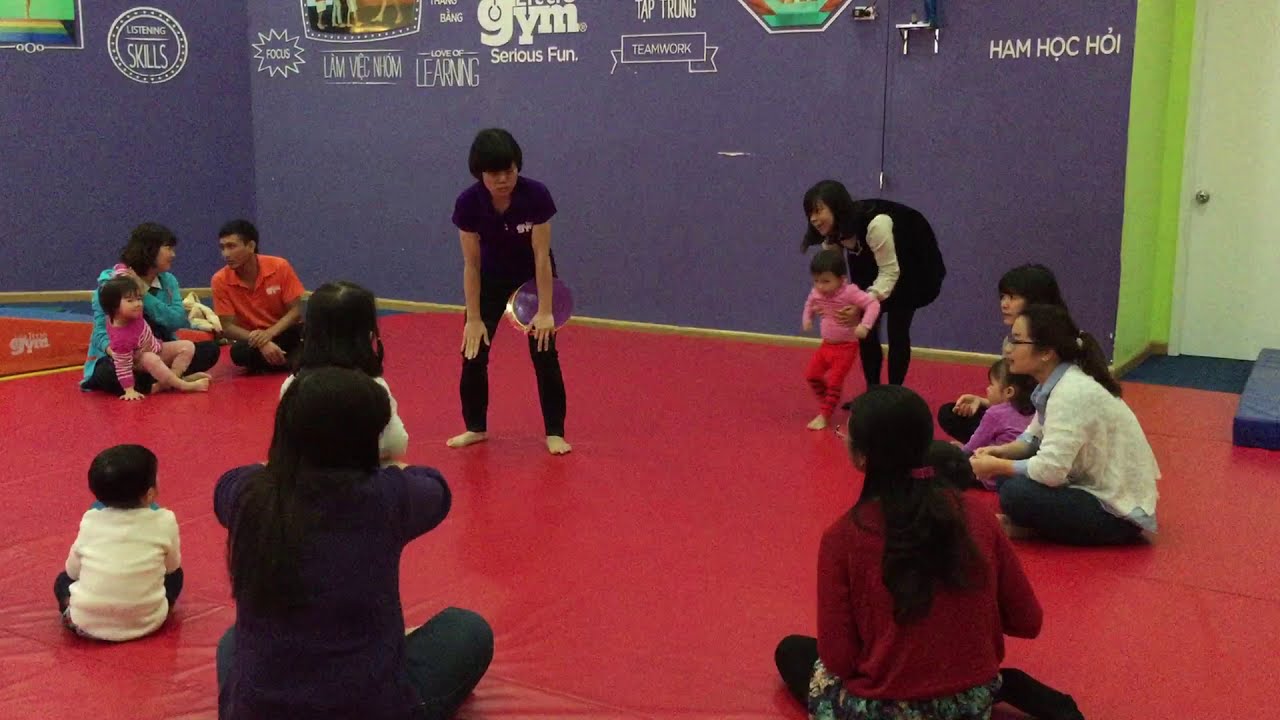The image showcases a lively scene inside a large gymnasium with padded red flooring, which appears to be a lively, indoor learning center decorated with numerous white logos on a blue wall, showcasing phrases such as "listening skills," "focus," "love of learning," "serious fun," and "teamwork." In the focal area, about five to seven parents, predominantly mothers, along with some fathers, are arranged in a circular formation, engaged in an activity. They are holding their children, indicating a family-oriented session. Most participants are seated on the red cushion matting, while a few are standing or squatting. At the center, a barefoot instructor, holding discs or purple plates, demonstrates a pose with their hands on their knees, suggesting an interactive fitness or educational session. In the top left, a man and a woman engage in conversation with a child. To the right, a woman in a black dress with a white undershirt holds a child clad in pink. Various children and adults exhibit diverse postures and attire, creating a warm, bustling environment highlighted by additional elements like a white door with a silver handle on the blue wall and a distinct blue step on the far right. The vivid colors and detailed logos emphasize the center's focus on combining physical activity with developmental skills in a supportive, family-inclusive setting.